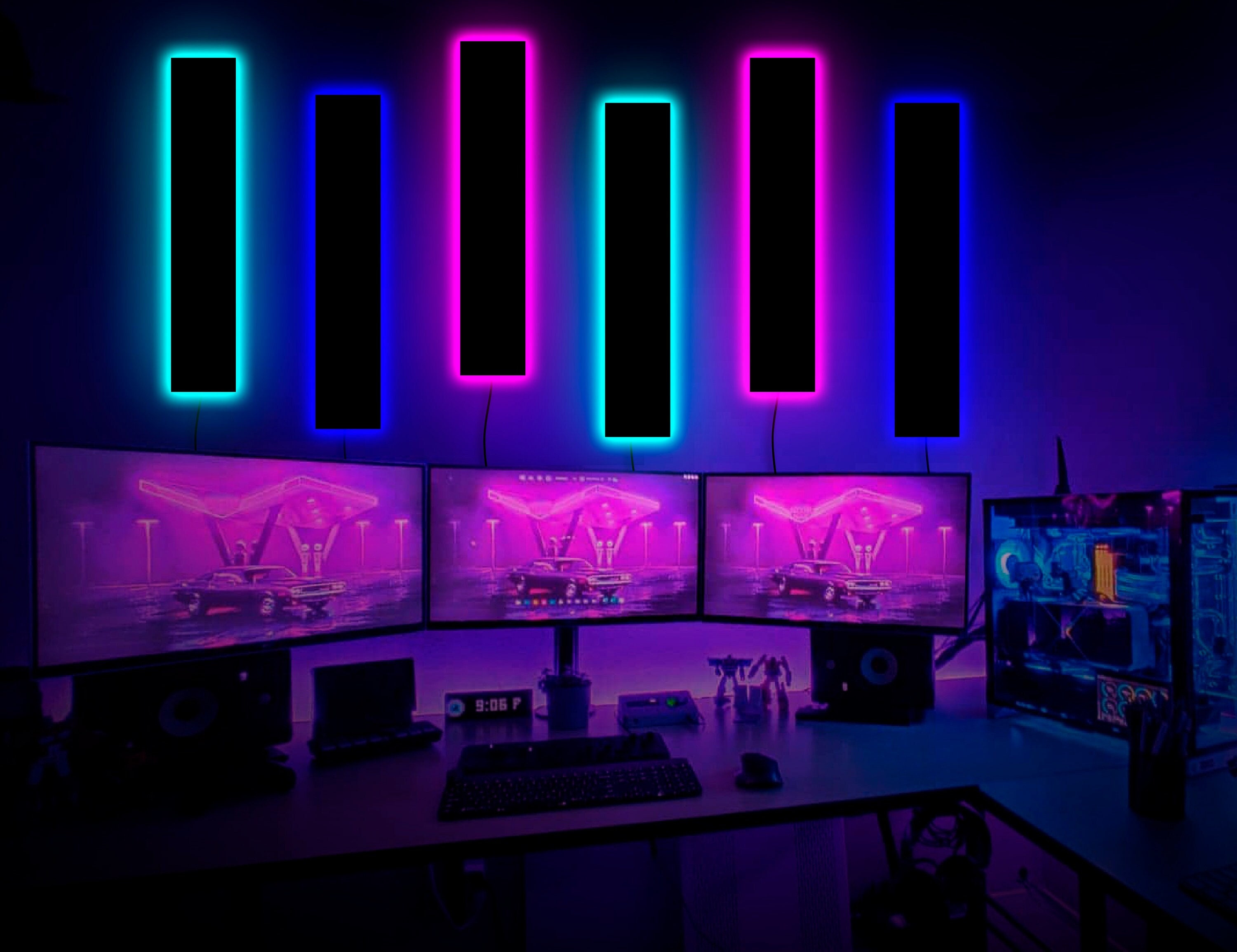The image depicts a dimly lit game room exuding a cool, almost otherworldly blue glow. The ambient lighting is provided by six narrow, rectangular neon lights mounted on the wall. These lights sequence from left to right in colors: aqua, blue, pink, aqua, pink, and blue. The glow from these lights reflects off the wall, creating an immersive gaming atmosphere. The centerpiece of the room is an L-shaped desk arranged with three large computer monitors, each displaying the identical image of a car parked in front of what appears to be a 1960s-style drive-up restaurant with a distinct pink neon glow, reminiscent of classic diner aesthetics. Below the monitors sit speakers, providing an enhanced audio experience. On the desk, there's a small digital clock displaying the time as 9:06, an ergonomic mouse, and a keyboard. Adding to the gaming ambiance, to the right of the setup is a blue glowing object that could be the main computer system. The desk also features two action figures resembling transformers and a pair of headphones tucked underneath. This array of high-tech and nostalgic elements suggests a competitive gaming setup designed for immersive experiences.